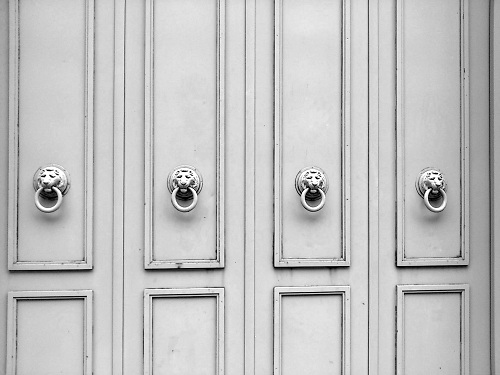This black and white photograph captures an intricate, decorative wall featuring four tall, rectangular door panels arranged side by side. Each panel has framed sections at the top and bottom, giving the wall a sophisticated wainscoting appearance. The doors are painted a very pale grey, almost blending into a white and pristine backdrop, which makes it difficult to discern, but they are likely made of wood. The most striking feature of the doors are the lion head door knockers, which appear to be made of either silver or a tarnished brass or gold metal. Each lion head holds a ring in its mouth, forming the knocker. The metal's aged look adds a sense of patina and character to the scene, while slightly dirty or damaged areas along the door panels enhance the photograph's textured detail. The repeated lion heads provide a focal point against the restrained, elegant backdrop of the wall.